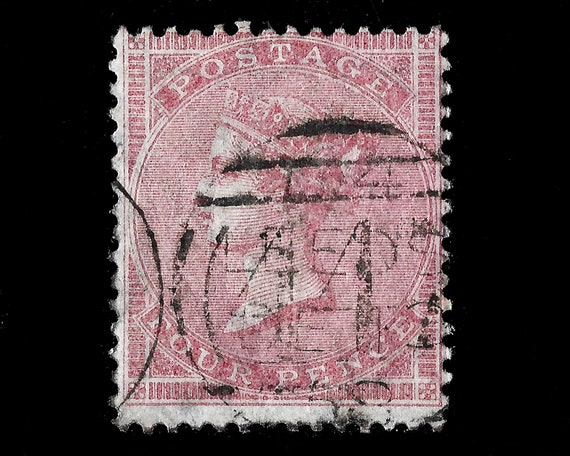This photograph features a vintage British stamp, primarily in a pinkish-red hue, with a rectangular geometric border. The central design showcases an etched silhouette of a woman, presumably a queen, adorned with a medieval-style crown, depicted in profile from the neck upwards. Above the circular portrait, the word "POSTAGE" is arched in a serif font, while the denomination "FOUR PENCE" is inscribed at the bottom in matching typeface. The stamp is heavily postmarked in black, with a circular imprint reading "LEADS" and some additional, illegible text. The background of the image is predominantly black, highlighting the detailed and intricate design of the aged stamp.